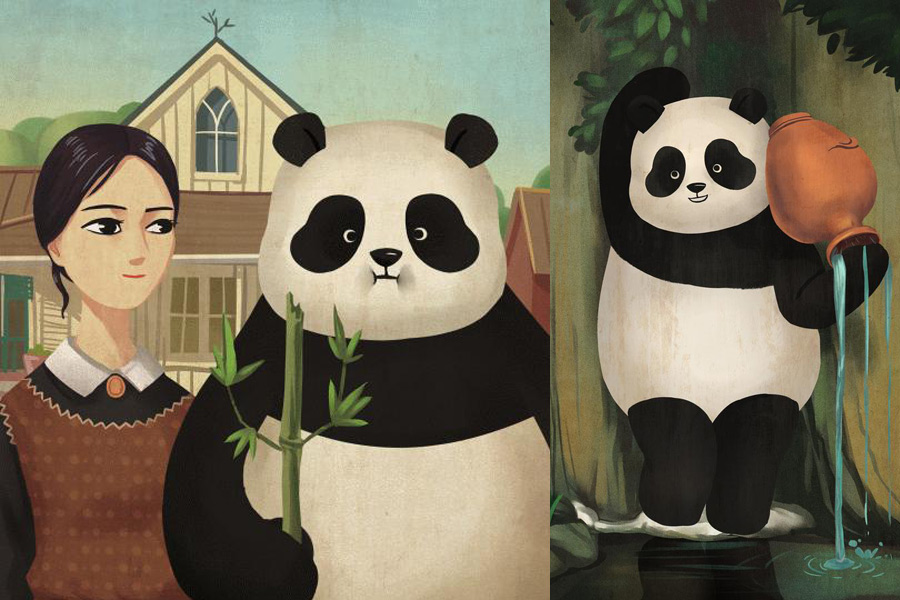The image consists of two side-by-side paintings featuring panda bears. 

On the right, there's a detailed painting of a panda bear with a white head and distinctive black markings around its eyes, ears, nose, neck, and legs. It carries an orange bucket over its shoulder, from which blue liquid spills, splashing onto the ground. Surrounding the panda are lush green leaves and vegetation, and the panda's other paw is raised above its head, giving an impression of being at a water's edge among the trees.

The left painting resembles the classic American Gothic artwork but with a whimsical twist. A panda bear stands in place of the farmer, holding a piece of bamboo positioned like a pitchfork, with leaves curling up on both sides. The panda has a white head with black ears and black eye patches, extending down to its nose and neck, while its arms are also black. Next to the panda, a woman with dark hair tied back in a ponytail and large, cartoonish eyes stands. She wears a brown dress with a zigzag edge, a light brown shirt with a white collar, and an orange cameo pin. She gazes straight ahead, completing the homage to the iconic painting. Behind them, an arched-roof house and some trees dot the background.

Both paintings, rich in detail, juxtapose traditional art with playful, panda-inspired reinterpretations.